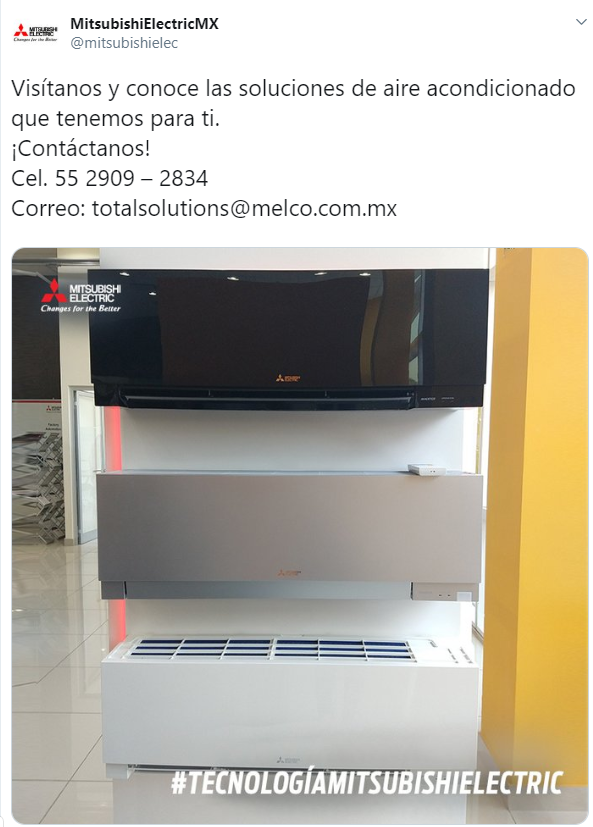The image showcases three different air conditioning units from Mitsubishi Electric, prominently centered and displayed vertically against a backdrop. The top unit is sleek and black, the middle one is a darker matte gray, and the bottom unit is a pristine white. To the right, there's a gold-colored column, and to the left, tile flooring continues into another section, giving a showroom-like setting. The red Mitsubishi Electric logo, with its distinctive three-petaled design, is located in the top left corner. The accompanying text reads "Mitsubishi Electric, changes for the better," followed by the hashtag "Technologia Mitsubishi Electric." Additionally, the image appears to be part of a tweet from Mitsubishi Electric MX, instructing viewers in Spanish to contact them via cell number 552-909-2834 or email at totalsolutions@melco.com.mx for more information.